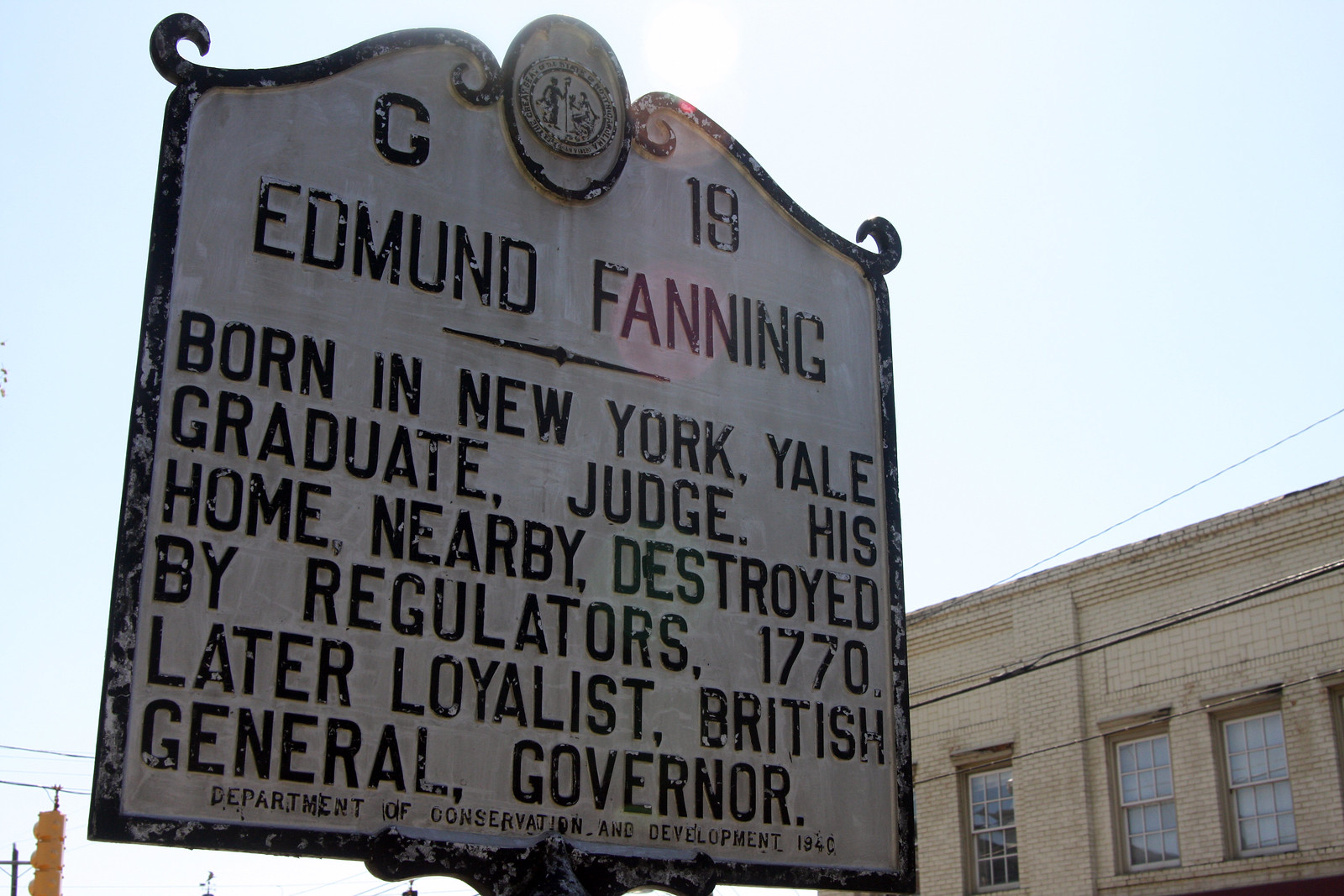The photograph depicts an outdoor scene during the daytime, featuring a historic marker prominently placed to the left. The marker, made of white metal with black lettering, bears the label "C-18" alongside an oval medallion, possibly a state seal. The sign reads: "Edmund Fanning, born in New York, Yale graduate, judge. His home nearby destroyed by regulators, 1770, later loyalist, British General Governor." Below this text, in smaller letters, it notes, "Department of Conservation and Development, 1940." Behind the sign is an off-white brick building with a few visible windows. To the left of the sign, traffic wires stretch across the view, and a yellow traffic light can be spotted. The scene is devoid of people, suggesting a quiet moment captured in a potentially historic district in the United States.